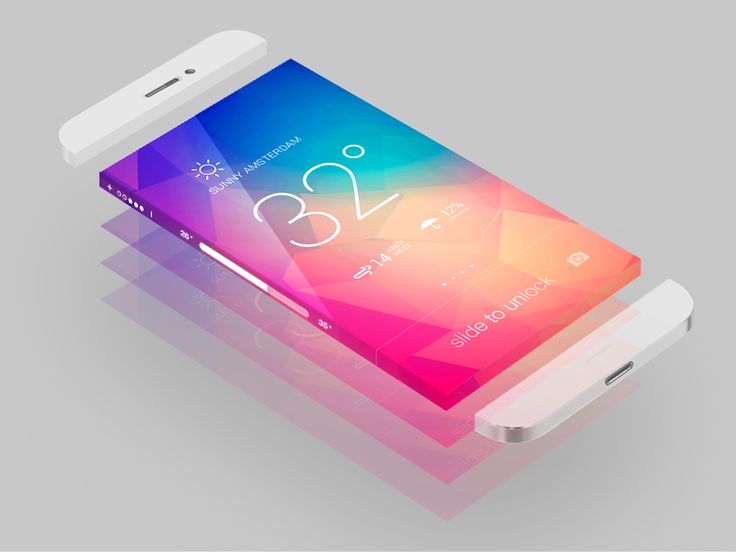This is a detailed, artistic digital illustration of a white iPhone depicted in three disassembled parts set against a gray background. The top section features the front camera and speaker, the middle section contains the vibrant, multicolored screen displaying weather information for Amsterdam, and the bottom section includes the charging port area. The screen showcases a blue, orange, and pink geometric wallpaper with a temperature of 32 degrees, an image of the sun indicating sunny weather, and additional weather details such as a wind speed of 14 and a 12% chance of rain represented by an umbrella icon. The interface includes 'Slide to Unlock' and a small camera icon. The side of the phone also displays a volume button. Each layer of the screen is intricately detailed, giving the impression of depth as they descend toward the bottom of the image.